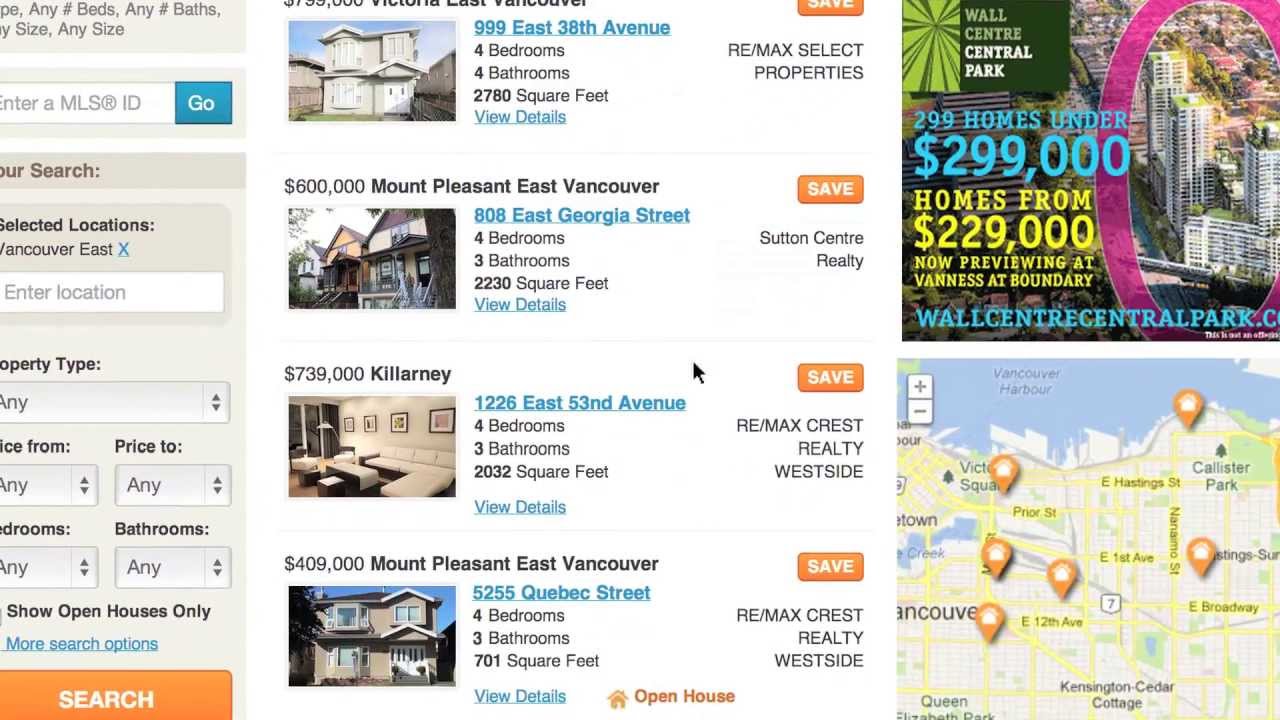This screenshot from a real estate website features a listing of four houses, primarily two stories and priced at $400,000 and up. Detailed information includes:

1. The first house.
2. The second house in Mount Pleasant, East Vancouver, priced at $600,000.
3. The third house located at 10226 East 53rd Avenue in Killarney, listed for $739,000. It boasts four bedrooms and three bathrooms.
4. The fourth property at 5255 Quebec Street in Mount Pleasant, East Vancouver, priced at $4,900, is indicated as an open house.

Each property listing includes an orange 'save' button. At the bottom right, a small map insert displays five orange markers showing the locations of the listed houses. Above this map is an ad banner from Wall Centre Central Park promoting 209 homes priced under $299,000, with options starting at $229,000.

On the left pane of the screen, a detailed filter section allows users to sort properties by type, price, number of bedrooms, and bathrooms. It also includes an option to display only open houses and the capacity to search using an MLS ID number, with a search button highlighted in orange at the bottom.